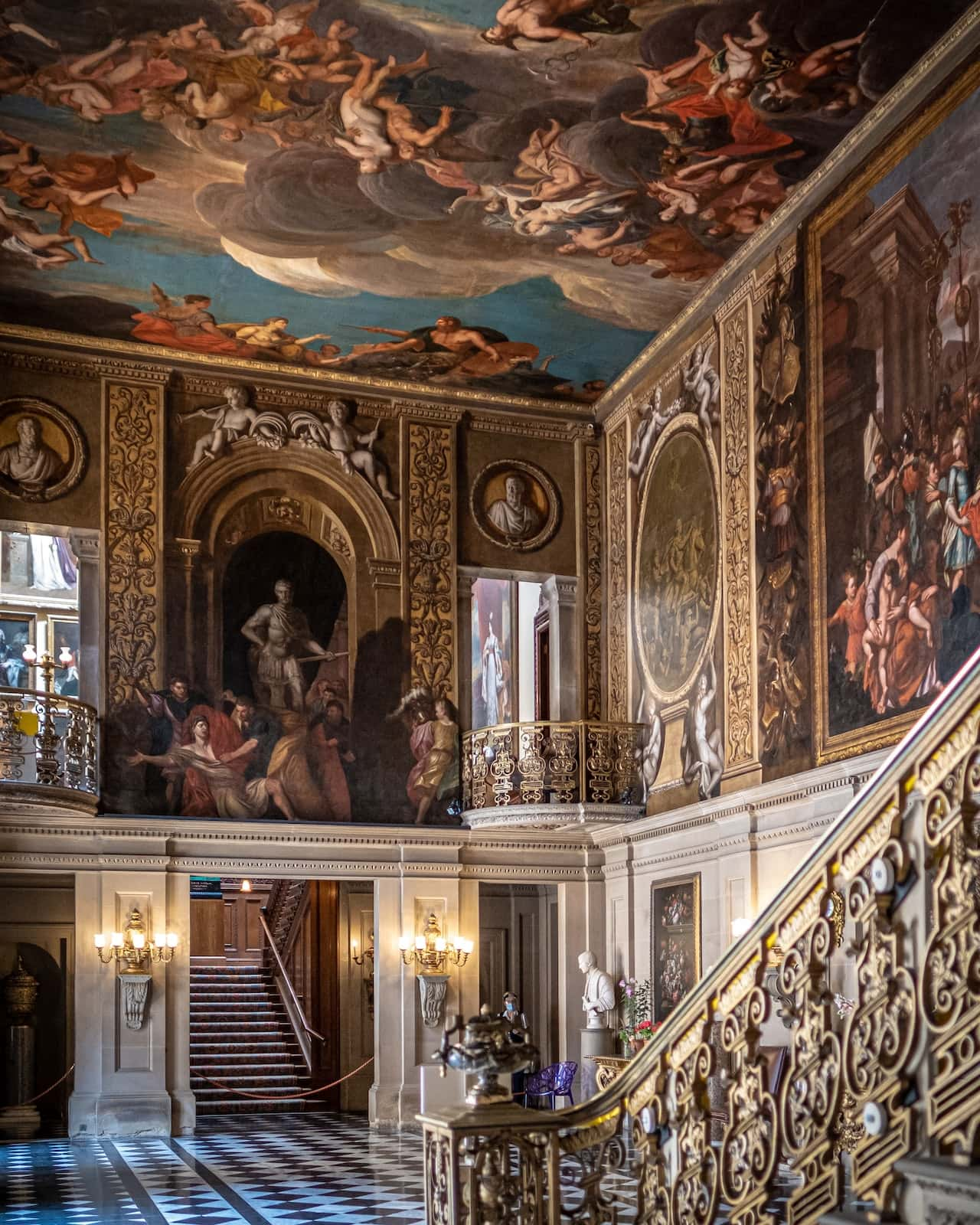The photograph depicts the opulent interior of a grand stately home or a museum, showcasing its richly ornate decor. Dominating the space are floor-to-ceiling frescoes, resplendent with religious and classical figures, drawing parallels to famed Renaissance works like those by Raphael. The frescoes, in hues of red, blue, brown, and yellow, extend to the elaborately painted ceiling, contributing to the room's lavish aesthetic. Brass balconies adorned with intricate designs overlook the scene, with the second floor visible through doors that reveal an art gallery hung with paintings. Central to the image is a marble and wood grand staircase, perhaps crafted from brass and pewter, complemented by parquet checkered marble flooring. Old-style wall lights cast a warm glow, further highlighting the room's gold accents and muted tones. This sumptuously decorated space, indicative of European influences, is steeped in history and artistry.